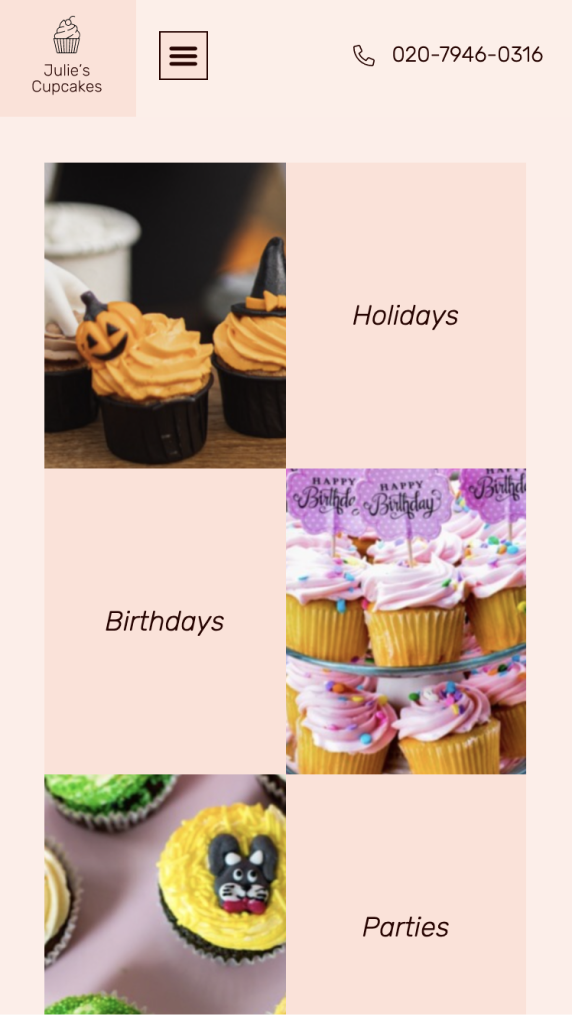This is a detailed screenshot for Julie's Cupcakes, a business specializing in gourmet cupcakes. In the top left corner, there is an elegant line drawing of a cupcake above the company's name, "Julie's Cupcakes." On the top right, a telephone receiver icon is displayed alongside the contact number: 020-7946-0316. 

The screenshot features several sections highlighting their offerings. The first section includes a photograph of two cupcakes perfect for the holiday season. The cupcake on the left is adorned with vibrant orange frosting and a small decoration featuring a jack-o-lantern. The one on the right mirrors the Halloween theme with orange frosting topped with a miniature witch's hat. The word "Holidays" is prominently displayed next to this festive image.

Beneath this, there is an image of a double-tiered tray filled with beautifully decorated cupcakes. The cupcakes seem to be made from yellow cake and are topped with light pink frosting and colorful sprinkles. Those on the top tier are also embellished with toothpicks holding purple, cloud-shaped signs that read "Happy Birthday." The word "Birthdays" is positioned next to this celebratory display.

To the right, there is another photograph featuring cupcakes ideal for parties. One standout cupcake is topped with yellow frosting and a cute icon of a dog. Additional cupcakes, partially visible in the background, are decorated with contrasting yellow and green frosting. The label "Parties" is located beside this playful array.

The screenshot encapsulates the diverse and creative cupcake options available at Julie's Cupcakes for various occasions.